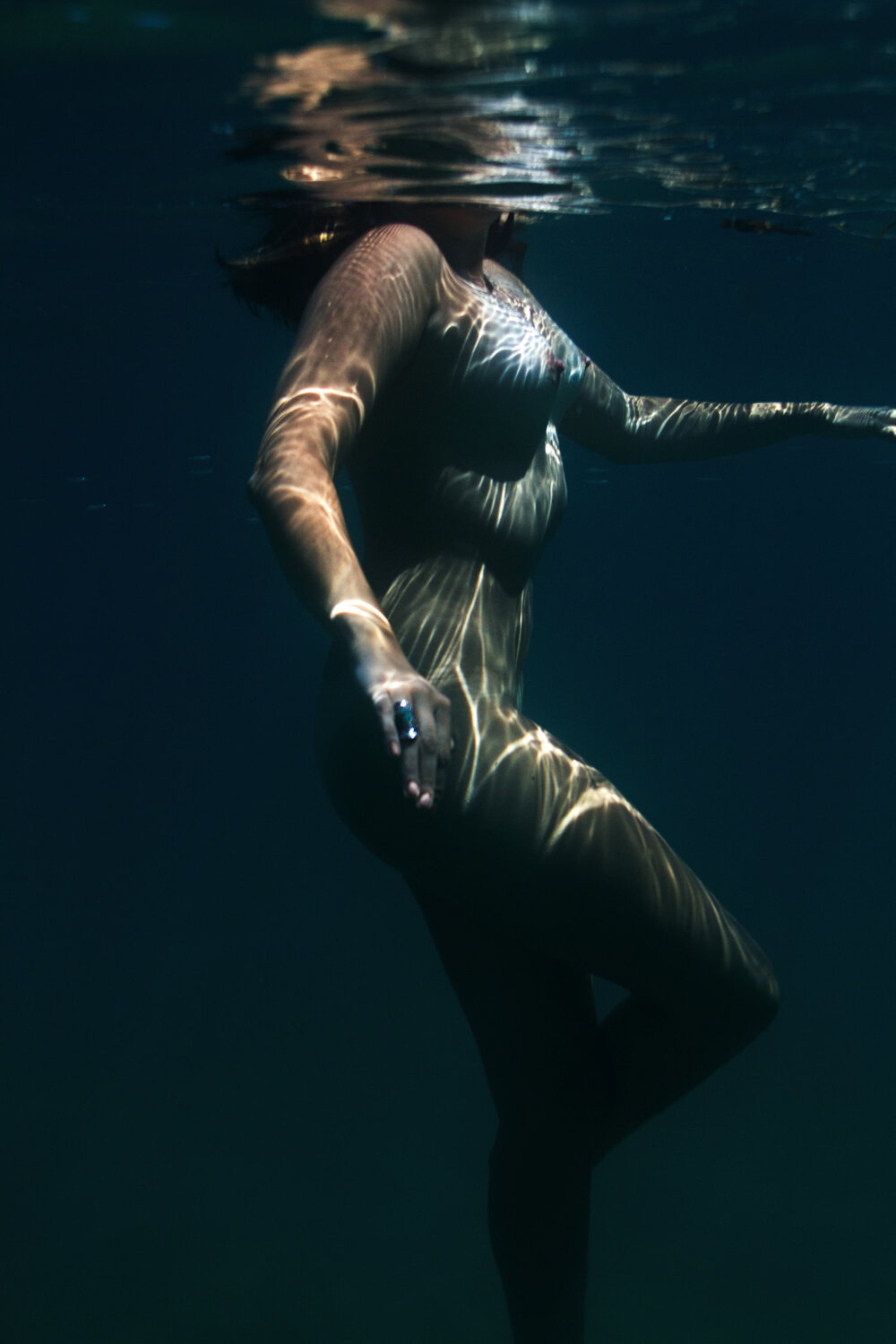The image captures a nude woman submerged underwater, with her head just above the surface, creating a slightly blurred reflection. The scene is set against a dark backdrop, with her body illuminated by the refracted light that creates mesmerizing patterns across her skin. She has long hair that gently floats in the water, accentuating the serene atmosphere. The woman is standing on the bottom of a swimming pool, facing her right, with her left arm extended perpendicular to her body and her right arm resting by her side. Adorned on her right ring finger is a prominent ring featuring a blue stone set in either gold or silver. Her left leg bears her weight while her right leg is elegantly bent over the left. The water’s surface at her neck height forms soft waves, enhancing the image’s tranquil and ethereal quality.